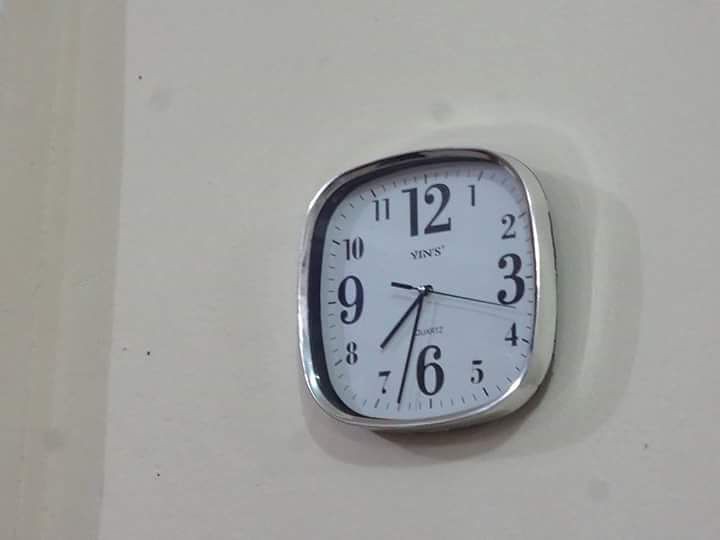This indoor photograph features a square-shaped clock with rounded corners, mounted on a plain off-white wall. The clock's sleek, chrome edges gleam under the lighting, casting a double reflection shadow due to multiple light sources in the room. Its black hands—the second hand, minute hand, and hour hand—are set to 7:33 and 17 seconds. The numerals on the clock face are designed with the numbers 12, 3, 6, and 9 larger than the others, creating a distinctive visual emphasis. The brand name "YINS" is prominently displayed near the top, with the word "quartz" situated above the number 6.